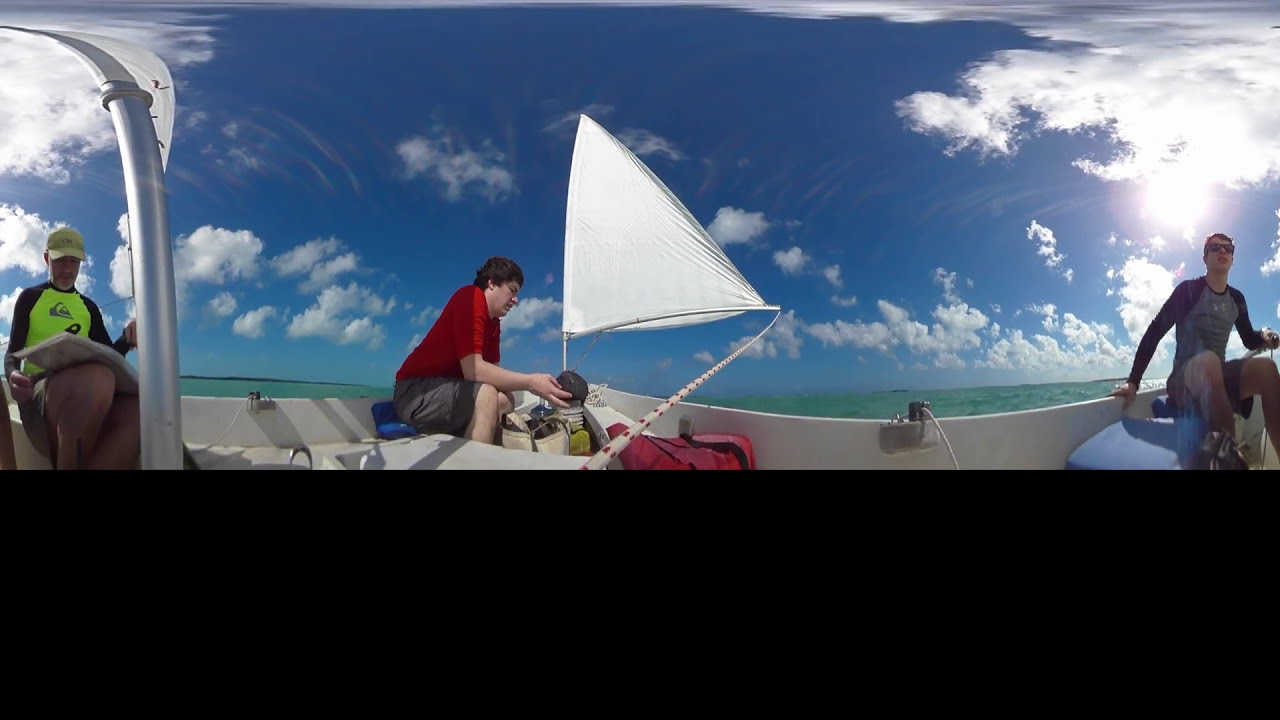In this vivid outdoor scene aboard a small sailboat, the expansive, deeply blue sky is dotted with numerous white clouds, with the bright sun peeking out from behind a cloud in the upper right. The boat features a somewhat distorted perspective, possibly due to a fish-eye lens. To the very left, a man dressed in a neon yellow and black shirt and matching hat is seen looking down, perhaps at a piece of paper or a map. Centrally positioned and sitting down, another man in a red shirt and gray shorts is holding an object in his right hand that resembles a large rock or coconut. Dominating the middle of the image is a large white sail with a white rope speckled with red dots. The background water showcases a greenish hue. On the far right, a man with a gray shirt and long blue sleeves sits on a blue seat, wearing black sunglasses. The entire scene, set against a backdrop of endless sky and ocean, suggests a bright midday adventure at sea.